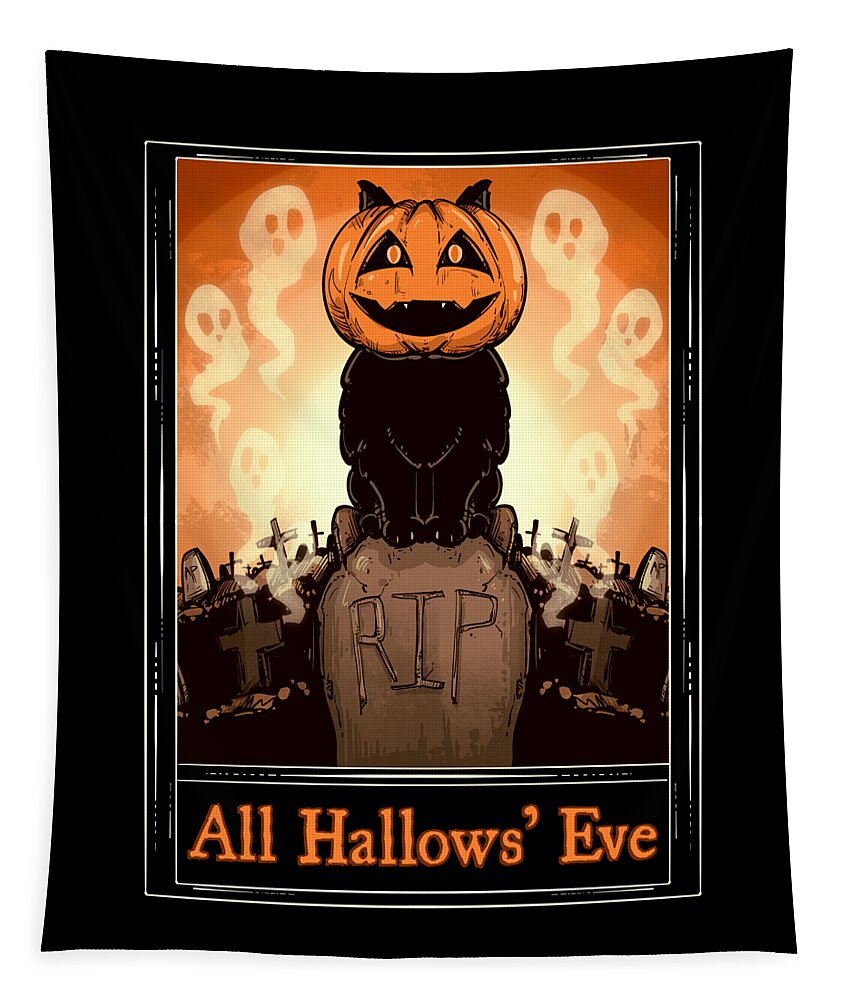The image is a color illustration framed by a thick black border. At the center is a Halloween scene with a graveyard backdrop, primarily in grays and blacks, contrasted by an orange background and white elements. A central tombstone, marked "R.I.P.," serves as a pedestal for a black cat. Unique to the scene, the cat wears a jack-o'-lantern over its head, with its ears poking out and its orange eyes visible through the triangular openings of the pumpkin. Adding to the eerie atmosphere, three white, squiggly, tadpole-shaped ghosts hover on either side of the tombstone. Surrounding the central elements are numerous other gravestones, some in the shape of traditional headstones and others as crosses. At the bottom of the image, the text "All Hallows' Eve" is written in orange, completing this detailed Halloween depiction.